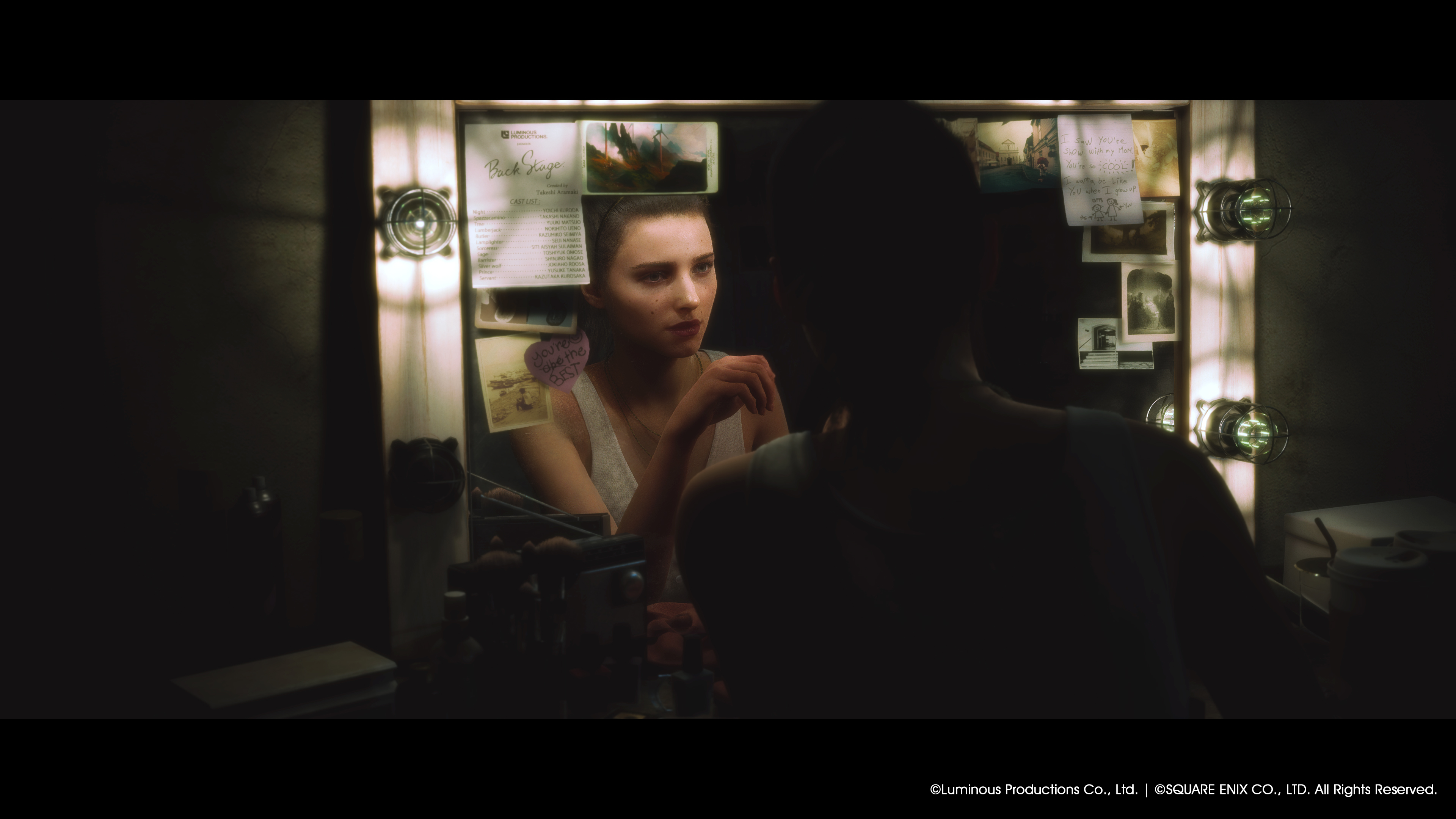In this detailed scene from a video game, a girl is depicted in her bedroom, sitting on a chair and looking into a mirror directly in front of her. The mirror is surrounded by various items, including notes, photographs, and multiple light bulbs, adding to the intricate and personal ambiance. The colors in this setting include beige, a light purplish-pink hue, and light green tones. The girl, who is wearing a sleeveless shirt, seems to be lost in thought as she gazes into the mirror. At the bottom right of the image, the text "Luminous Productions Co Ltd. Square Enix Co. Ltd. All rights reserved" is clearly displayed, indicating the production companies behind this evocative visual.